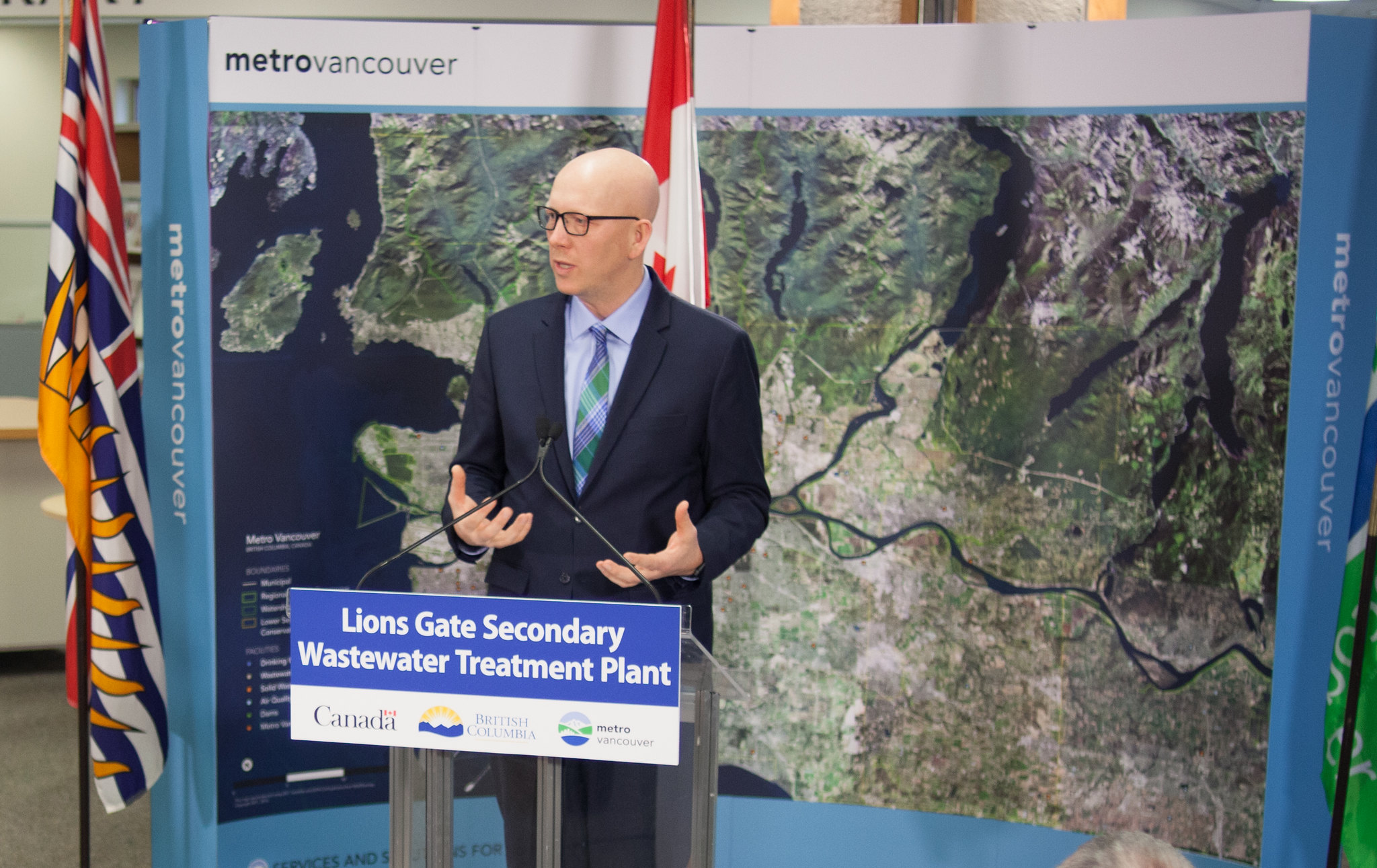A bald man with dark-framed glasses stands before a movable stage setup, speaking into two microphones mounted on a plastic podium. He is dressed in a dark blue suit, a light blue shirt, and a blue and green checkered tie. Behind him is the sign for the Lions Gate Secondary Wastewater Treatment Plant, featuring a white text on a blue background with a horizontal white band below that includes the word "Canada." To the right, part of a Canadian flag is visible, and to the left, a colorful flag with red, blue, white, and an orange sun can be seen, albeit flopping downward. A large map labeled "Metro Vancouver" is displayed in the background.